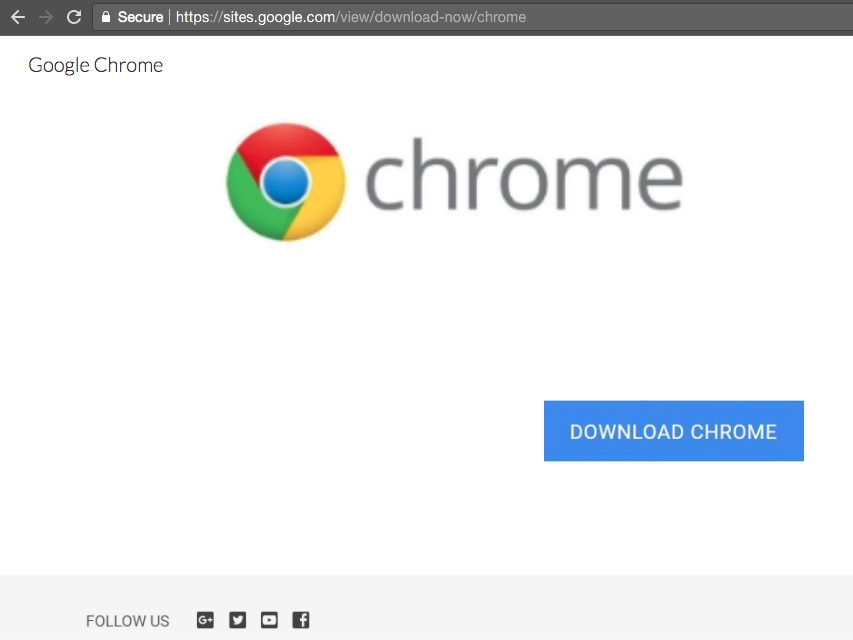This image, sourced from a website, features a predominantly black background at the top, with navigational icons including a white arrow pointing to the left, a dark arrow pointing to the right, and a refresh circle icon. The URL is prominently displayed: https://sites.google.com/view/download/now/chrome.

Transitioning to a white background below, the image features the title "Google Chrome" in black text aligned to the left at the top. Centered on the page is the word "CHROME," also in black text, accompanied by the Chrome logo to its left—a blue circle surrounded by red, yellow, and green segments. Beneath this, aligned to the right, is a blue rectangular button with the text "Download Chrome" in white.

At the bottom right corner of the image, there is a "Follow Us" section, featuring icons for Google+, Twitter, YouTube, and Facebook, inviting users to follow Google Chrome on these social media platforms.